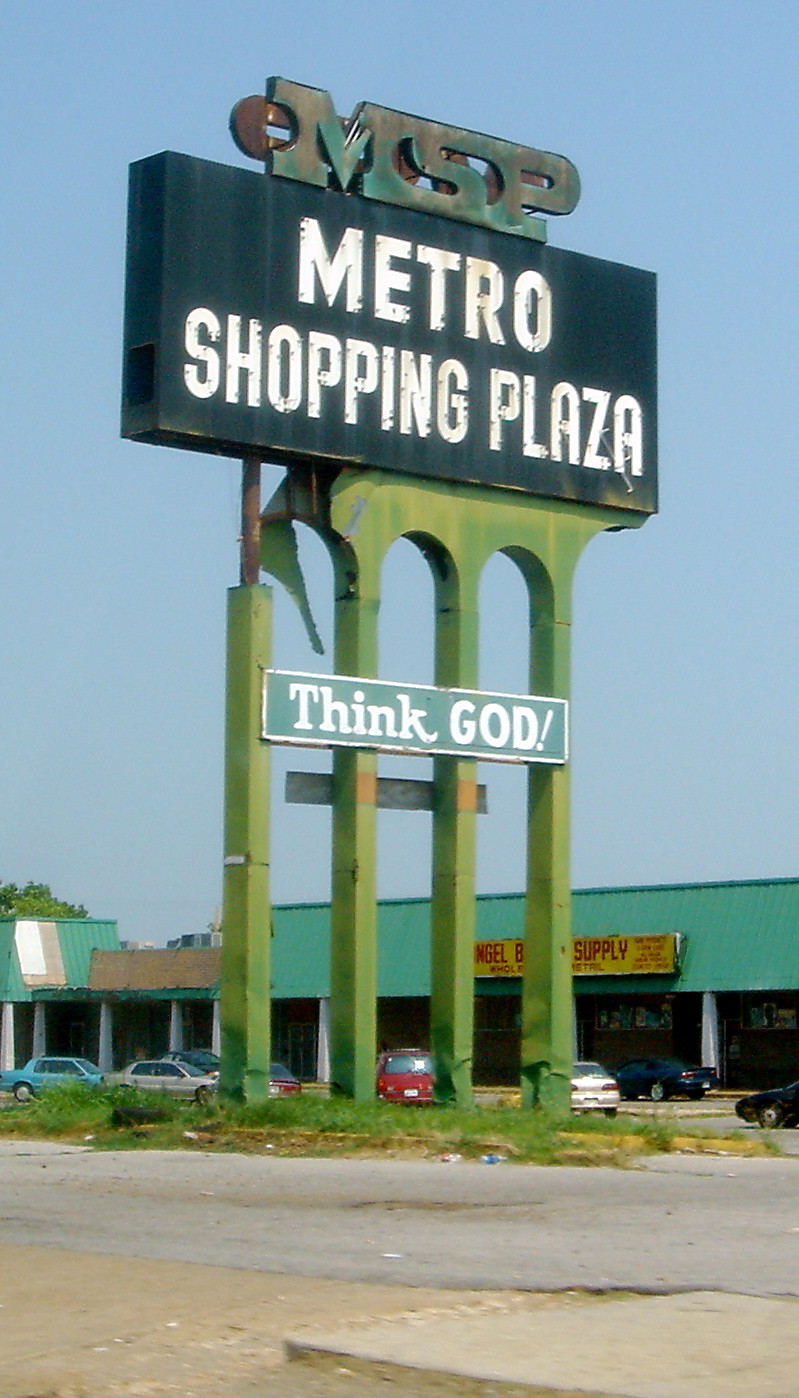This photograph captures a street-side sign taken from a viewpoint across the street, possibly from a parking lot. The sign, supported by four green pillars that form three arches, appears to be deteriorating at the top, suggesting the metal pillars are covered by light green paper. The rectangular sign, dark green and landscape in orientation, prominently displays "Metro Shopping Plaza" in white letters. Above this, the abbreviation "MSP" is written in green letters. The sign stands adjacent to a shopping center with a noticeable green roof. Nearby, a partially visible yellow sign with red lettering reads "Something Supply." Several cars populate the parking lot, and across the street, a concrete sidewalk is visible.